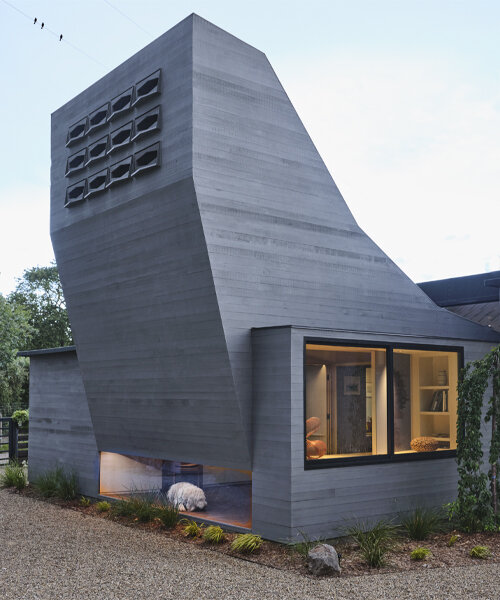This photograph showcases a very modern, abstract-designed house composed predominantly of gray concrete. The base of the structure is a rectangular prism, featuring two large glass windows on its right side that reveal a room with a blue door and a white bookcase. Above the base, a peculiar, polygonal shape juts out and angles back, resembling a rubber chicken, adding an unconventional flair to the building's architecture. The middle section houses a brightly lit, orange-tinged window through which various items can be seen. Positioned beneath this strange polygonal section is a gravel yard with small plants and a white dog peacefully sleeping. The background of the image features a faint light blue sky with white clouds and lush green trees, enhancing the modern yet organic ambiance of the scene. Additionally, an array of vents is noticeable on the side of the polygonal structure, emphasizing its unique and functional design elements.